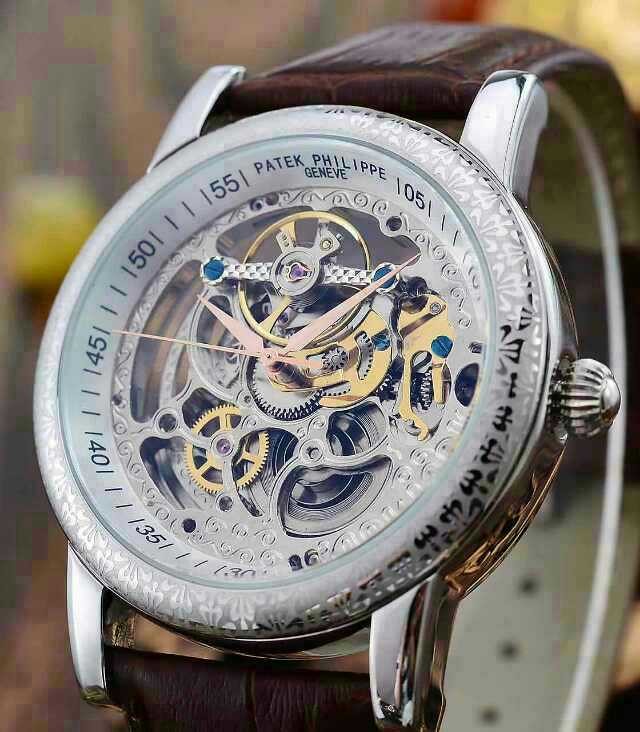This close-up image showcases an intricate and expensive wristwatch distinguished by its transparency, revealing the complex inner workings of its mechanics. The silver frame encircles a marvelous display of intricate gears, some crafted from regular steel, copper, and gold-colored components, adding to the richness and elegance of the design. The hour, minute, and second hands are a light rose gold color and precisely indicate the time on an inner rim that bears the markings in intervals of 5—the numbers from 05 to 55, separated by minute lines. Notably, the hour numbers are absent, requiring careful observation of where the hands point.

The watch is emblazoned with the prestigious name "Patek Philippe Genève" at the 12 o'clock position, synonymous with European craftsmanship and luxury. The exterior features an ornate design, possibly an embossed logo that appears to resemble an E with an extended middle stroke. The opulence extends to the band, crafted from dark brown crocodile leather with a silver buckle, ensuring both comfort and sophistication. This meticulous masterpiece stands as a testament to the fusion of artistry and precision engineering.